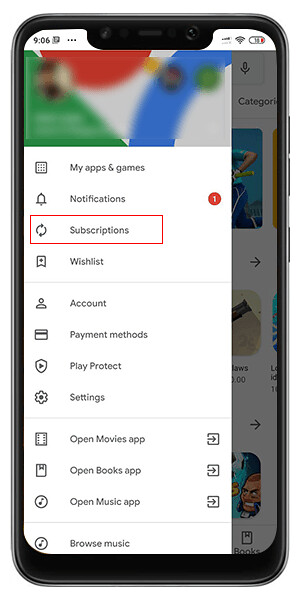The image features a front-facing digital representation of a smartphone screen displaying a detailed menu interface. The screen prominently shows a dropdown menu titled "My Apps & Games," which houses several sections. The first section includes items labeled "Notifications," with a red circle and the number "1" indicating a single unread notification, followed by "Subscriptions," and "Wish List." Below this, a small divider line separates these items from the next group of options: "Account," "Payment Methods," "Play Protect," and "Settings." Another divider line follows, leading to options for opening specific apps: "Open Movies.app," "Open Books.app," and "Open Music.app." At the very bottom, past one more divider line, there's an option labeled "Browse Music." In the background of the dropdown menu, faint images of app and game icons suggest that this menu is overlaid on an app store interface. Additional details include the time displayed as 9:06 and a low battery icon in the red zone, indicating that the phone needs charging.